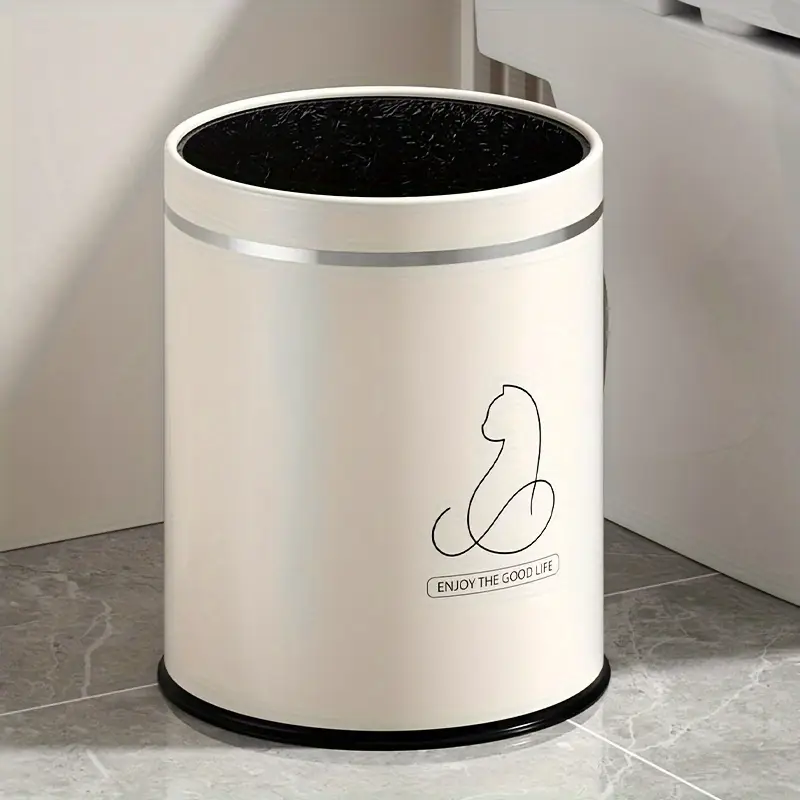The image depicts a small, cylindrical trash can placed on a gray, marbled tile floor within a kitchen or bathroom setting. The trash can is primarily white or cream-colored, featuring a thin black ring at the base and a silver band around the top. The interior of the can is black. Prominently displayed on the front is a simple stencil outline of a cat, accompanied by the phrase "Enjoy the Good Life." Positioned next to a white fixture and against a light cream-colored wall, the can exudes a minimalist yet playful aesthetic, fitting seamlessly into its surroundings.